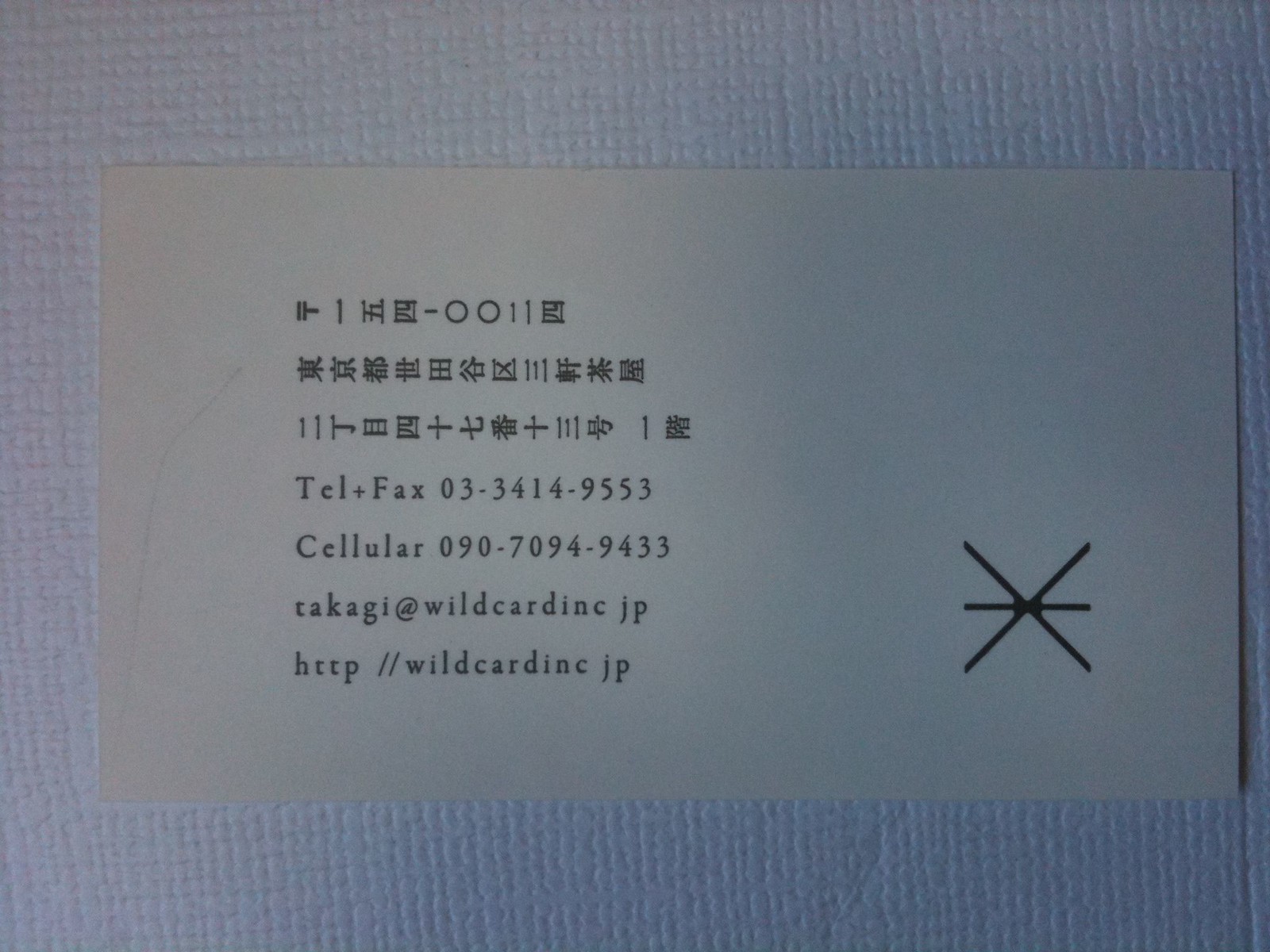The photograph showcases a business card placed on a white surface that features a slightly bumpy texture, noticeable through its small dots and lines. The business card, predominantly white, is centrally positioned in the image, occupying the majority of the composition. It displays a mixture of Chinese characters and English text spread across seven lines.

Starting from the top, the first three lines on the left side of the card contain Chinese lettering. Following these, there is a line that includes the words "Telephone & Fax" alongside a contact number. Beneath this, the term "Cellular" is listed with an additional phone number. An email address is written on the subsequent line, provided in English. At the very bottom of the card, there is a URL for a website, also in English.

The bottom right corner of the card features a distinctive logo consisting of three intersecting lines and two dots at the center. The overall design and the textual elements of the card stand out against the minimalistic yet textured backdrop.